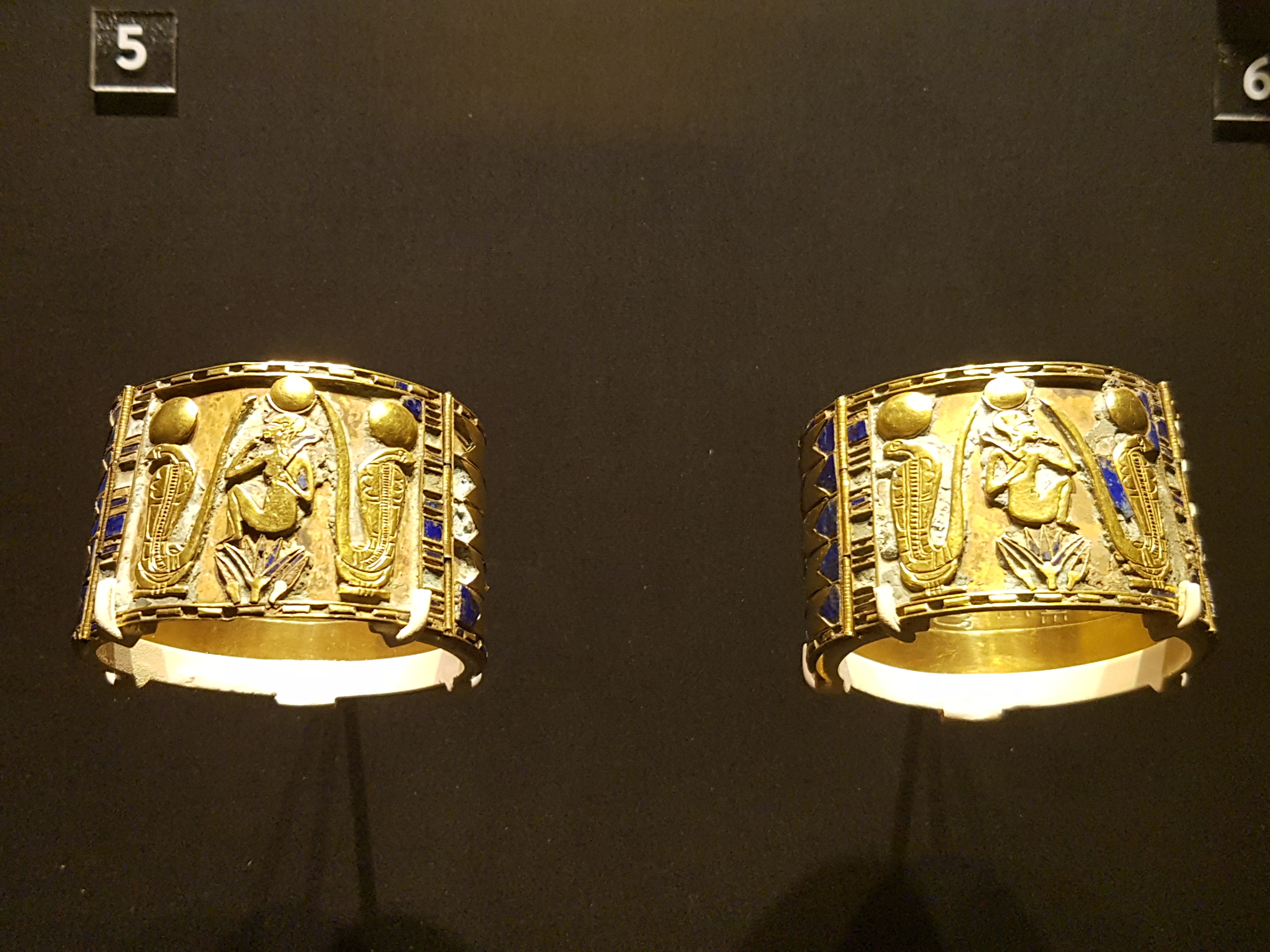The photograph captures a rectangular museum display with a black back wall. In the top left corner, a small black square placard bears the white number "5," while on the top right, another placard features the white number "6." Centered in the image are two ornate golden bangles adorned with intricate designs. Each bangle features triangular blue shapes and depicts an identical image of a person surrounded by two cobra snakes, although the image faces different directions on each bangle. The left bangle incorporates several blue squares to its left and right, whereas the right bangle showcases a row of five blue triangles with additional blue accents on the upper right and along the arch's rightmost part, suggestive of Ancient Egyptian aesthetics.